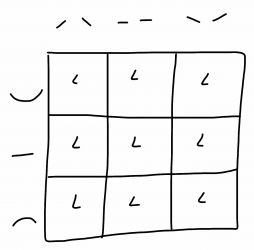The image appears to be a digital drawing produced on an iPad, possibly using an application like GoodNotes, and created with an Apple Pencil. The drawing consists of a large square that has been subdivided into nine equally-sized smaller squares, arranged in a 3x3 grid. Inside each of these smaller squares is a consistent small squiggle resembling a tiny "L". 

The top of the diagram has several horizontal lines serving as a form of navigation or separation. Down the left-hand side are three distinct navigational markers: the first row features a line that curves upward akin to a smile drawn on a stick figure's face; the second row displays a simple horizontal line resembling a minus sign; and the third row shows a line that curves downward like a frown on a stick figure.

The overall appearance suggests it could be a type of graph or tally chart, although no text accompanies the illustration to provide explicit context. The repeated motif of tiny "L" shapes within each square might symbolize data points or markers.